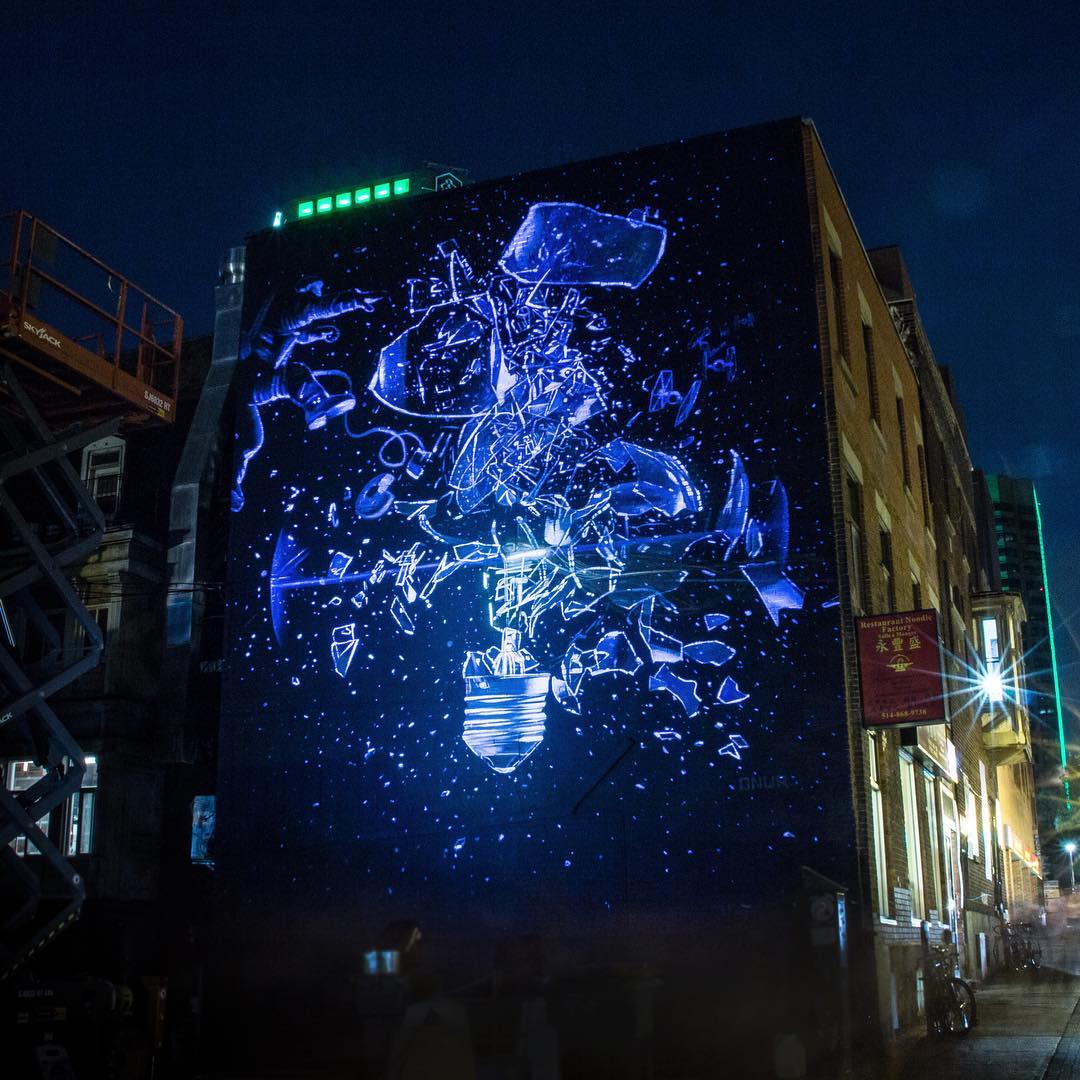This nighttime city street scene features a building adorned with a striking, illuminated piece of modern art. The three- or four-story brick and stone building, which appears to be older, is fronted by business signs and lights, with the side wall fully transformed into a dazzling canvas. A high-rise building and lit streets recede into the background, with a bike leaning against one of the buildings and a scissor lift positioned on the left side, suggesting recent or ongoing installation work.

The focal point of this image is a vibrant, multi-element projection on the building's side, dominated by shades of bright blue against a dark backdrop. The art depicts the bottom of a light bulb with the screw part clearly visible and appears to be shattered, with fragments resembling glass scattering outward. Among these chaotic shards are abstract humanoid figures and what appears to be astronauts floating amidst the debris, lending a surreal and trippy quality to the piece. Additional elements include large letters, notably an 'F' in the upper left corner, and swirling patterns evocative of stars and squiggles, all contributing to a night sky effect. The iridescent glow and intricate details make this an arresting and immersive display of contemporary artistry.